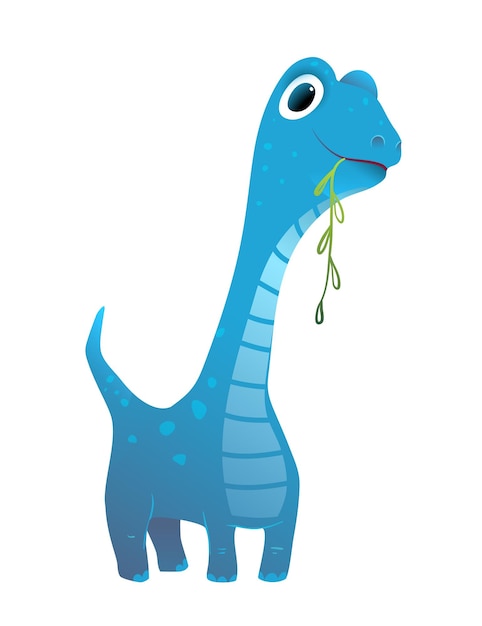The image features a whimsical, cute, cartoon blue dinosaur with a large bobble-head-like appearance, characterized by a very long neck and big eyes with prominent white and black detailing. The dinosaur has a cheerful demeanor, grinning with a green leafy branch hanging from the right side of its mouth. Its body, primarily a darker shade of blue, is adorned with lighter turquoise speckles, and its slightly short stature includes four legs and a small, upturned tail. The dinosaur’s chest showcases subtle lines, adding to its endearing, innocent look.